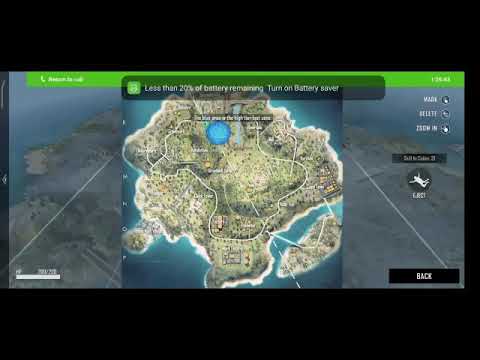This image is a detailed topographical map of an area, showcasing mostly green and yellow hues with a distinctive blue circle in the center, suggesting a body of water. White lines traverse the map, indicating pathways or roads. The top of the image features a prominent gray banner with a green square on one side, displaying the message: "Less than 20% of battery remaining. Turn on battery saver." Above this banner is another green bar. In the upper right corner, the numbers "134.43" are visible, alongside smaller, indistinct numbers. 

In the bottom right corner, there's a black rectangle with the word "BACK" printed in white, and above it is a dark circle containing an icon of a man with spread arms and bent knees, suggesting a descent as if parachuting. The image itself is bordered by a black rim, with the top and bottom edges being significantly thicker than the sides. The layout resembles a screenshot from a video game, potentially Fortnite, given the style and iconography, including features that suggest an interactive interface commonly found in game displays.